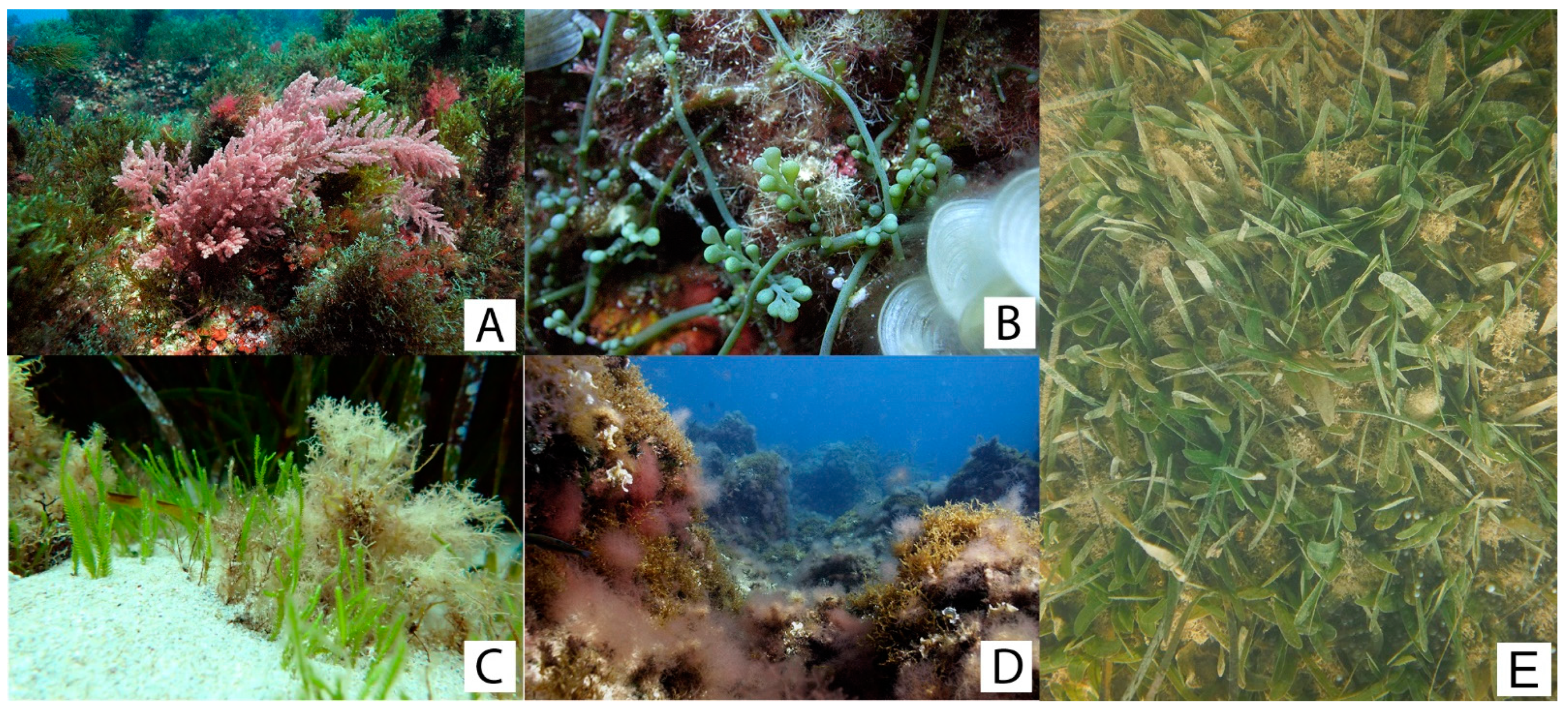This image consists of five distinct sections, each showcasing underwater scenes teeming with diverse marine plant life. Four of the sections, labeled A, B, C, and D, are of the same size and arranged in a grid on the left side. The fifth section, labeled E, spans the entire right-hand side and is roughly double the width of the others. 

In section A, the scene features vibrant pink corals amidst dense underwater greenery at the ocean floor. Section B provides a close-up view of green, pod-like plants intertwined with vines, and a translucent white object is noticeable in the corner. Section C captures grass-like stalks and additional ocean floor vegetation, with visible sandy patches. Section D portrays a coral reef area with rocky outcroppings adorned with marine plants.

Meanwhile, section E stands out as it might be interpreted as either an underwater or terrestrial environment, characterized by murky water and a mixture of green plants and beige grasses viewed from above. This detailed collage collectively highlights the rich variety of marine flora, primarily focusing on corals, sea plants, and other underwater vegetation.